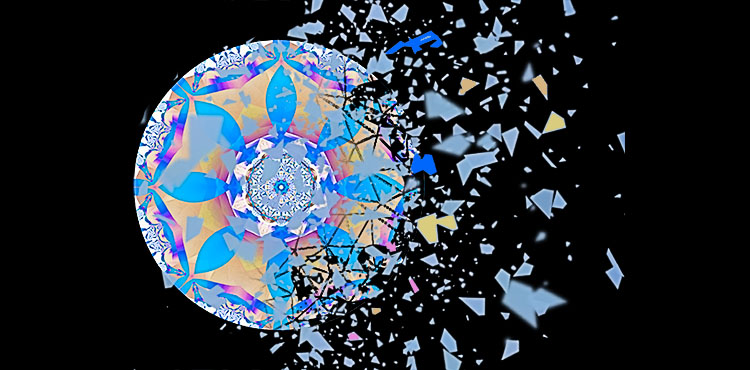The image depicts a digital animation styled as a kaleidoscopic design, set against a black background. At the center lies a circular pattern with concentric sections featuring an intricate mosaic of geometric shapes—an octagon surrounded by triangles—all radiating outward. The inner circle is filled with vibrant hues of blue, yellow, purple, and cream, while the outer sections also include shades of orange. Leaf-shaped blue shapes extend outward from the central pattern, adding depth to the overall design.

The composition evokes the impression of a shattered glass CD, with jagged shards flying off predominantly to the right side of the frame. These glass-like fragments, depicted in light blue, dark blue, yellow, brown, and pink, exhibit a dynamic sense of motion. Some of the closest shards appear blurry, as if too near the observer’s viewpoint to be sharply focused. Overall, the artwork combines a striking array of colors and shapes, with an illusion of breaking apart, conveying both beauty and disintegration in a single, cohesive image.